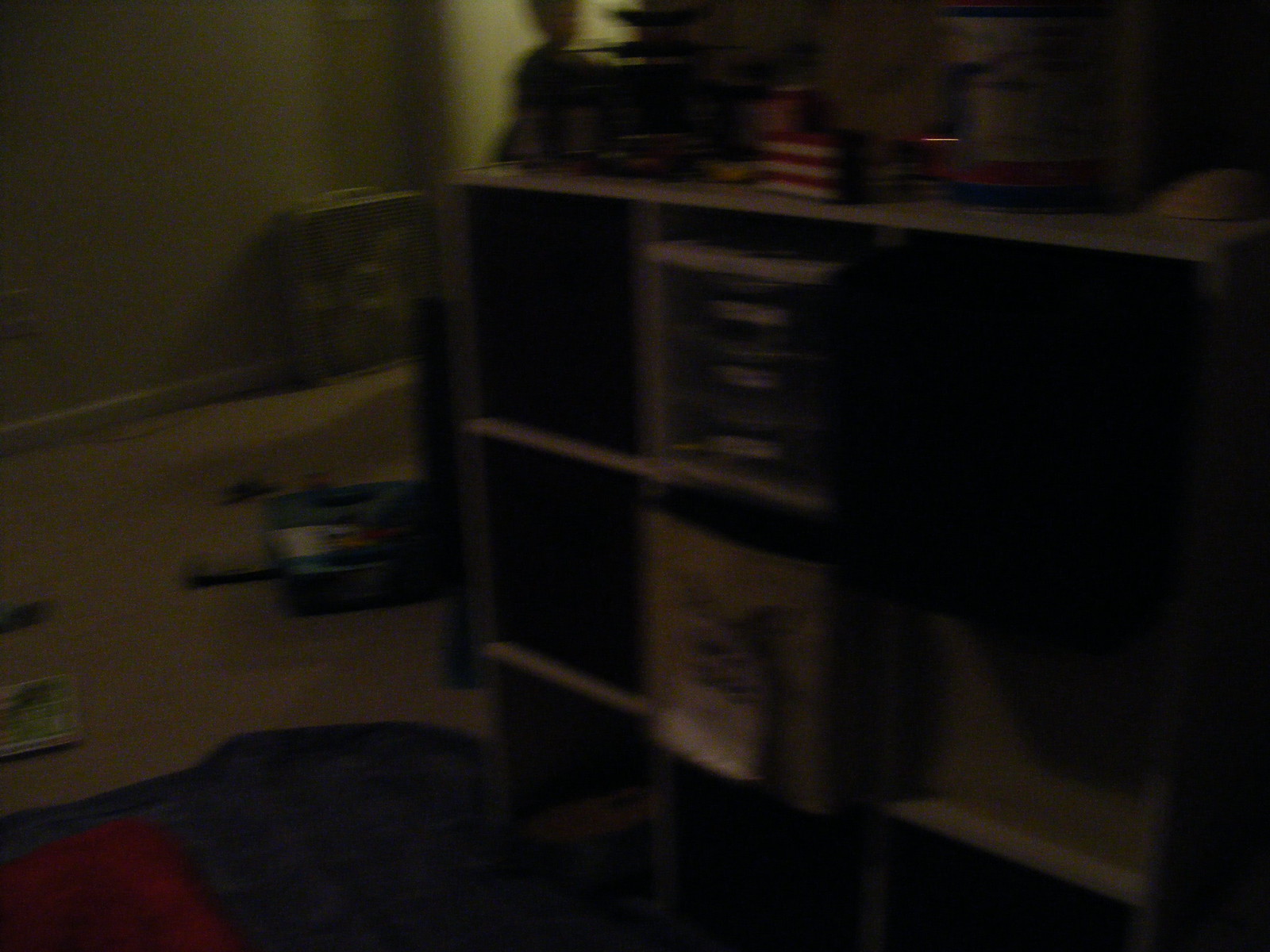In this dimly lit and blurry photograph, it is challenging to discern specific details due to the poor lighting and lack of focus. The setting appears to be someone's living room within a house or an apartment. A box fan, painted in a shade of light green, is positioned against the wall in the background. On a table in the foreground, there are several toys scattered across the surface. Beneath these toys, there seem to be two objects that could either be small microwaves or plastic trays typically used for holding office supplies such as pens and paper.